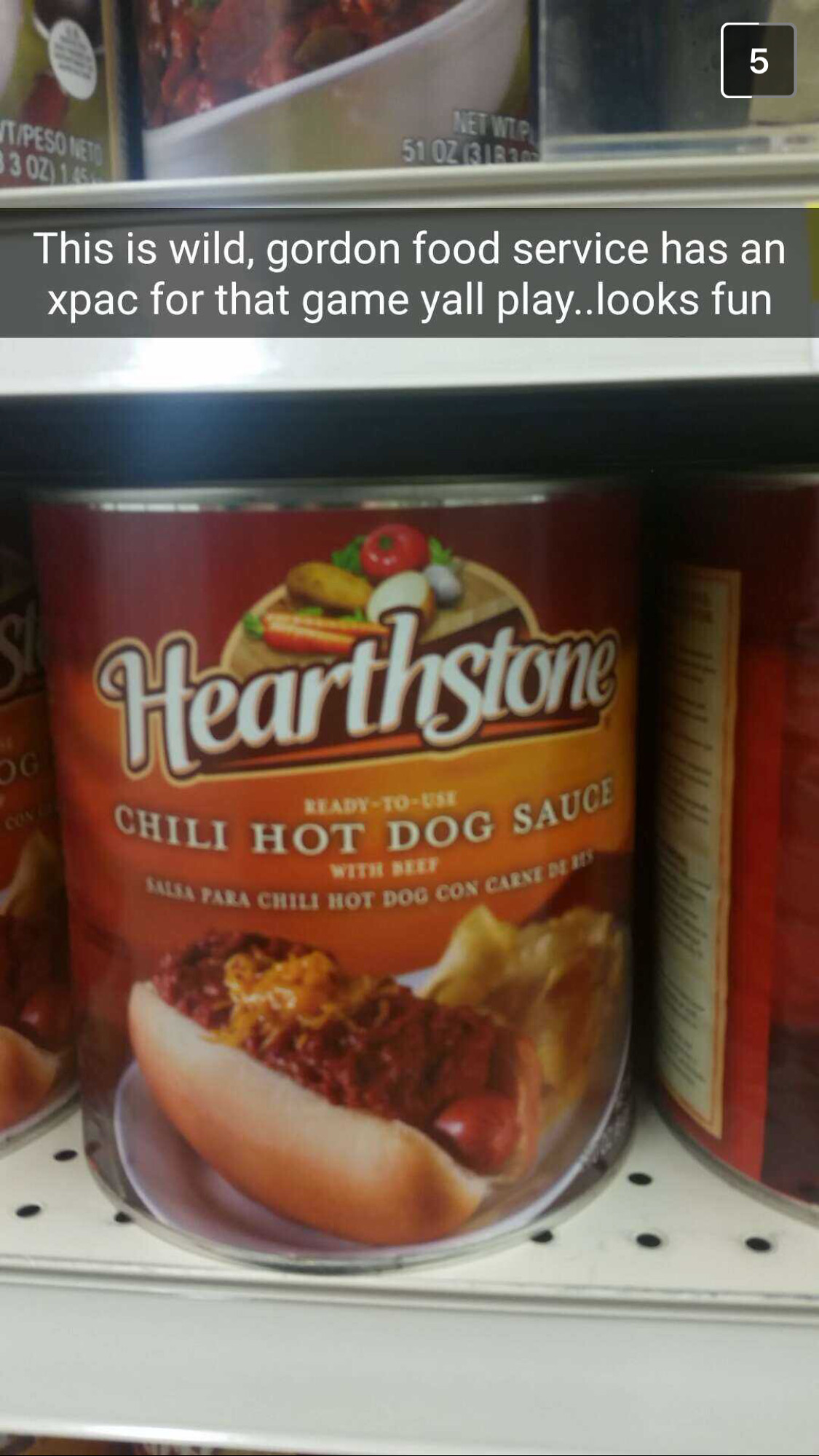This photograph captures a supermarket shelf, prominently featuring a can of Hearthstone brand ready-to-use chili hot dog sauce with beef. The can is red and orange, adorned with images of a hot dog topped with chili and cheese, alongside some potato chips. Above the brand name, illustrations of assorted vegetables—carrots, an onion, a potato, garlic, and a tomato—are displayed. 

The can's label includes both English and Spanish text, stating "chili hot dog sauce" and "salsa para chili hot dog con carne." The shelf is lined with multiple cans of the same product, arranged neatly. Above this image, the supermarket's gray shelf liner features a caption in white letters: "This is wild. Gordon Food Service has an x-pack for that game y'all play. Looks fun." Additionally, on the upper right of the image, the number 5 is inside a square frame, partly encircled by a white line.